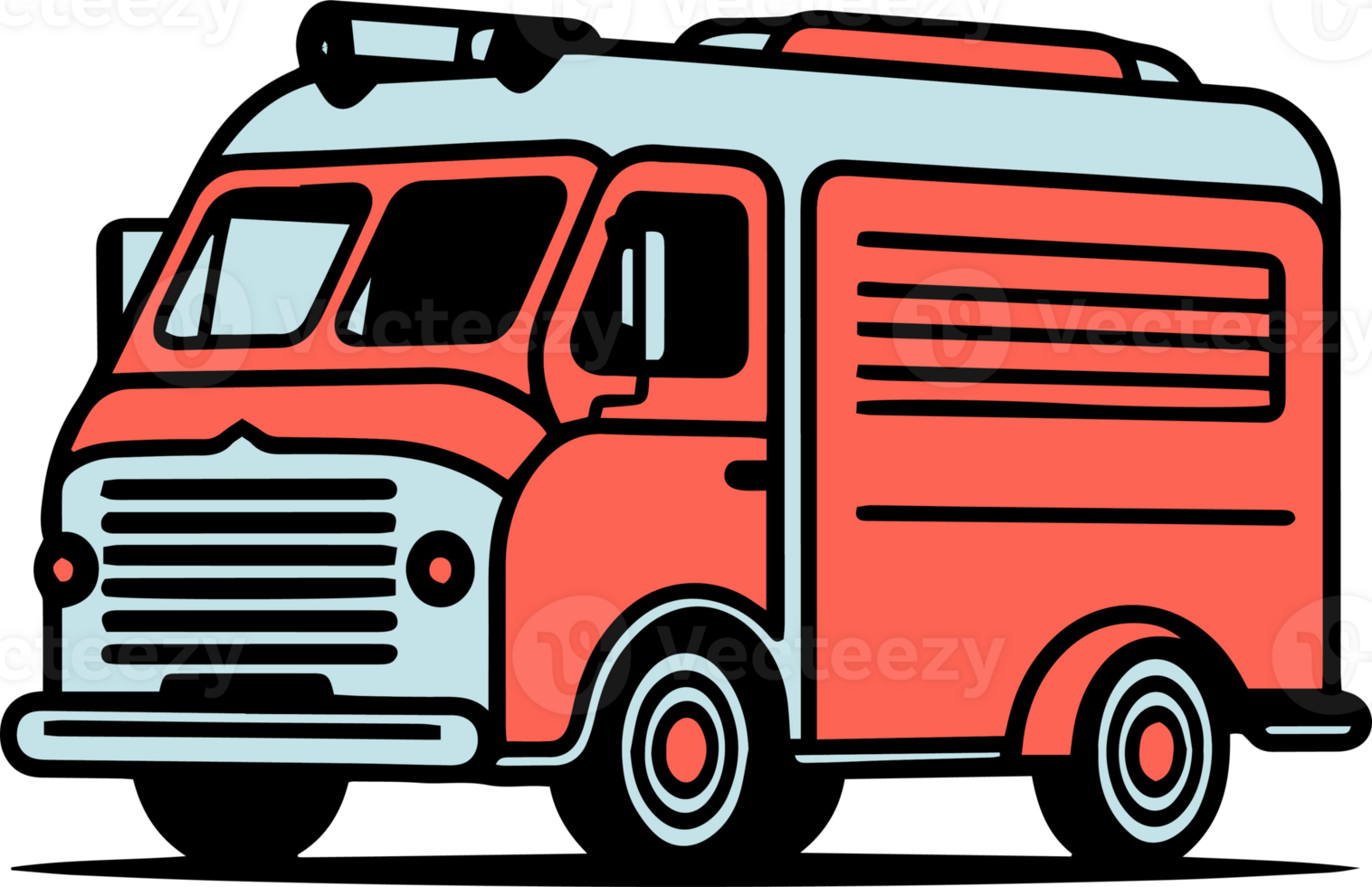This image is a cartoon-style illustration of a predominantly red truck or small service vehicle, possibly a firetruck or compact food truck, with gray and light blue accents. The truck is shown from a side angle, revealing its front and side profile along with two visible wheels. These wheels have a unique design featuring two blue circles with a red circle in the center. The vehicle is equipped with black, horizontal lines on its side and a gray bumper with a single black stripe.

The front of the truck features a gray grill with six horizontal gray lines and two red headlights encircled by black. There is a roof rack on top of the vehicle, and the cab area includes two windows: one for the driver and one for the passenger, each with an accompanying side mirror. The windshield is divided into two sections.

The image background is white with a faint watermark that seems to read "Vecteezy," and includes a "V" logo. The style of the illustration is simple yet detailed, with a noticeable shadow beneath the truck. This vibrant graphic, characterized by thick, black outlining, features no people or additional background elements.